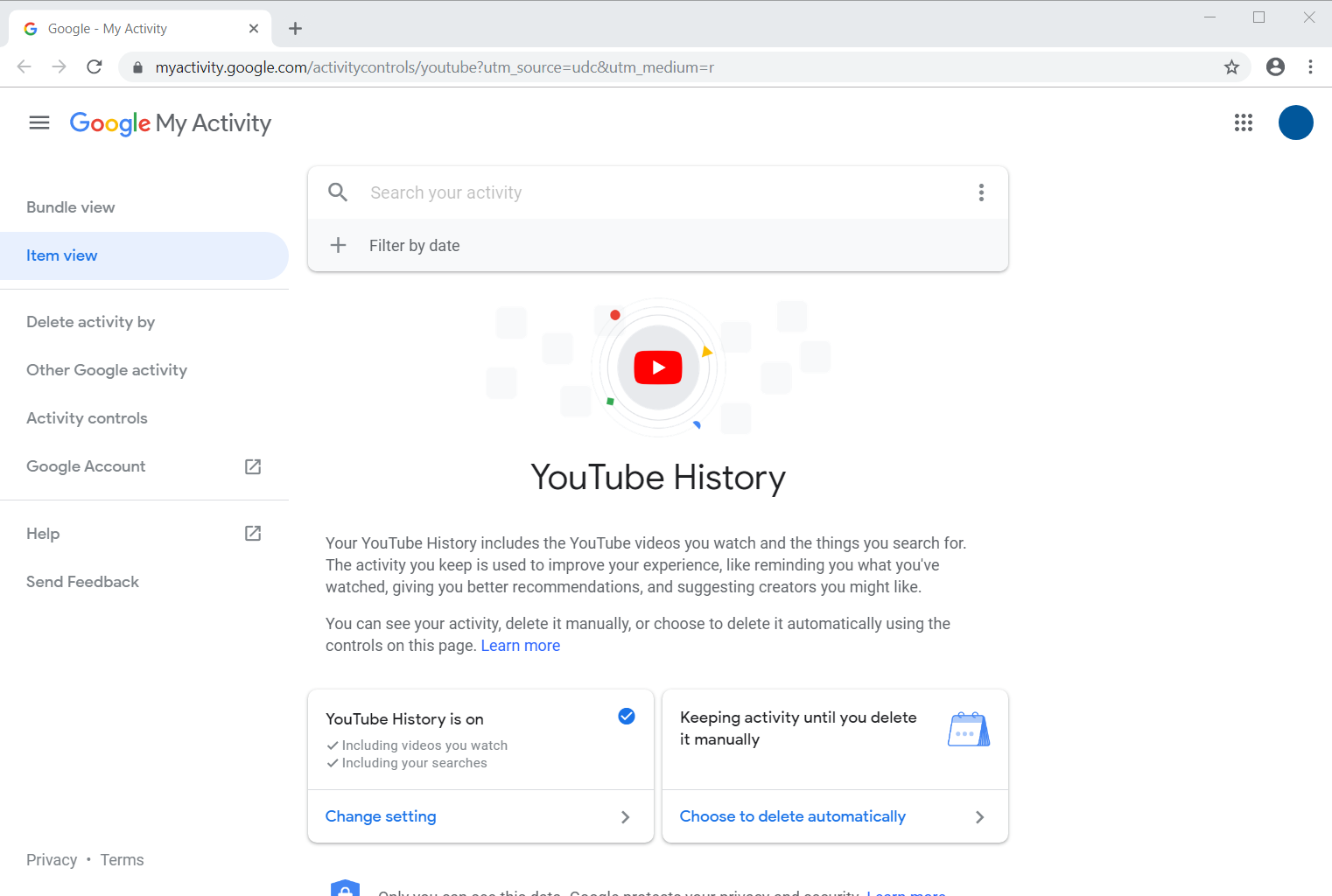This image is a detailed screenshot of a user's Google My Activity page. At the top of the screen, the browser's address bar is visible, indicating the URL for the My Activity website. 

On the left side of the screenshot, the Google logo is prominently displayed next to the title "My Activity." Below the logo, a navigation menu lists various options, including:

- **Bundle View**
- **Item View** (currently selected)
- **Delete Activity by**
- **Other Google Activity**
- **Activity Controls**
- **Google Account** (with a link that opens in a new tab)
- **Help** (also opens in a new tab)
- **Send Feedback**

Adjacent to the navigation menu, a search bar provides a function to "Search your activity," and includes filters for sorting results by date.

Further down the page, the YouTube logo (a red circle with a white triangle) appears, followed by a section detailing the user's YouTube history. This section explains that YouTube history includes both the videos watched and the search queries entered on YouTube. It emphasizes that the collected activity helps enhance user experience by reminding users of previously viewed content, offering better recommendations, and suggesting potential new creators to follow.

Below this explanation, a status message indicates that YouTube history is currently turned on. Users are informed that their activity will be retained until they choose to delete it manually, with options to modify these settings available via blue text links.